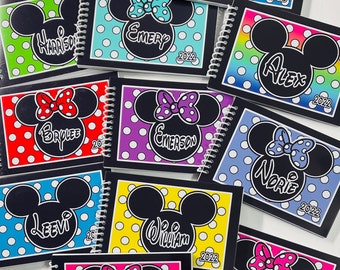The image captures an array of spiral notepads, each adorned with the iconic Mickey Mouse head in black, set against vibrant, polka-dotted backgrounds. The notepads feature an assortment of colors, including red, blue, yellow, purple, turquoise, lime green, and multicolored with white polka dots. Each Mickey Mouse head displays a name: Bailey is set on a red background with white stripes and polka dots, Levi on a blue background, William on a bright yellow background, Emerson on a purple background with a matching bow, Emery on a turquoise background, Nori on a powder blue background with a blue bow, Alex on a multicolored background, and Harrison on a lime green background. Additionally, there are parts of other notepads visible, including a pink one with a pink bow. The names are prominently written in white, sometimes outlined in black, positioned in the center of each Mickey Mouse head. Overall, the notepads form a colorful and playful arrangement reminiscent of the Mickey Mouse Club, emphasizing the classic Mouseketeer design.